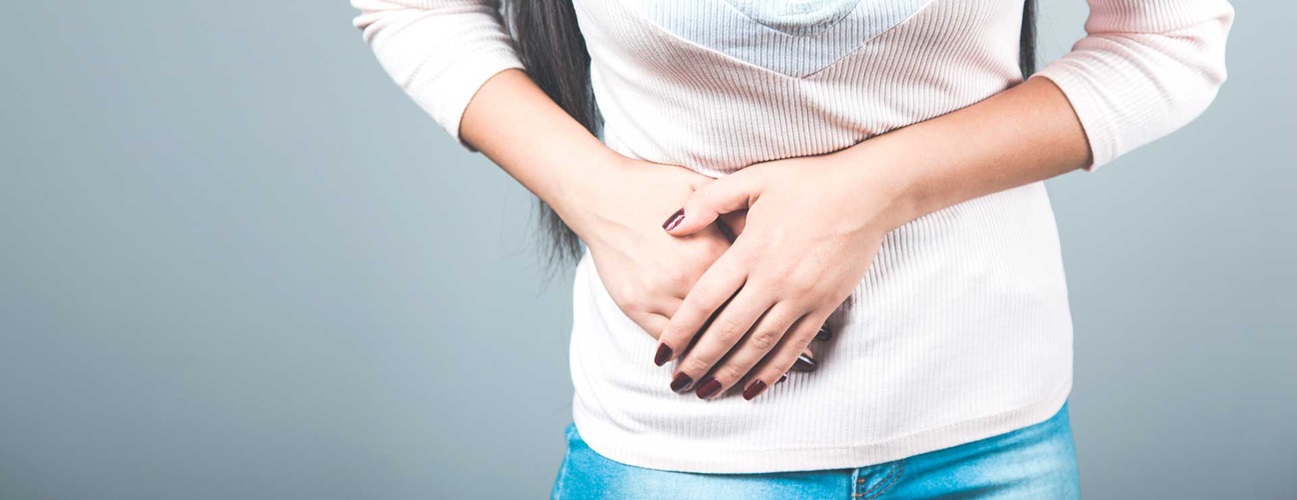This photograph captures the midsection of a woman standing in front of a light gray, reflective wall, suggesting a well-lit studio setting. She is wearing a ribbed, light pink, mid-sleeve top that extends past her waist, accompanied by faded, light blue jeans. Partially visible in the frame is her long, straight black hair, which cascades down to her waist. Her hands are crossed over her stomach, with her left hand resting on top of her right, indicating she might be experiencing stomach pain. Her fingers are adorned with deep wine or burgundy colored polish, adding a detailed touch to her medium-toned skin. The veins on the back of her hands are slightly pronounced, emphasizing the tension in her posture. She stands oriented towards the right side of the image, conveying a sense of discomfort.